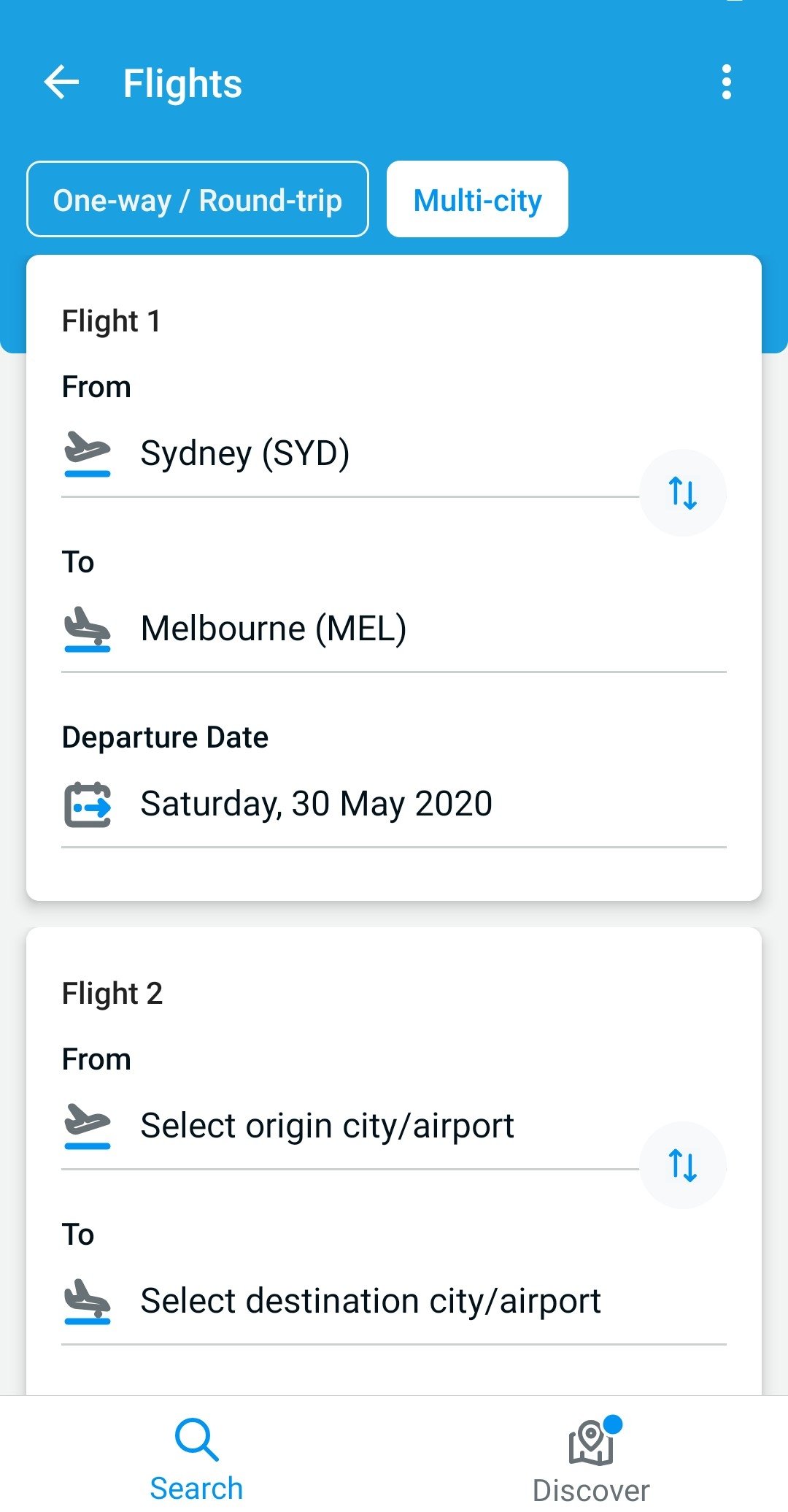This image features a webpage designed for booking airline flights. At the top, there's a prominent blue rectangle with "Flights" written in white letters located in the top left corner, accompanied by an arrow pointing to the left. On the right-hand corner of this blue section, there are three dots arranged vertically.

Directly below this header, users can choose between "One-Way," "Round-Trip," and "Multi-City," with "Multi-City" currently highlighted in white text against a blue background. 

The next section contains a blue square labeled "Flight 1." This area allows users to specify their journey details. It includes fields for the departure city, symbolized by an airplane icon, which currently reads "Sydney (SYD)," and the destination city, also denoted by an airplane icon, listed as "Melbourne (MEL)."

Further down, there is a departure date field that when clicked, opens a calendar. For this specific itinerary, the departure date is set to "Saturday, 30 May 2020." 

Following this, there is an option to add details for another flight segment. This area, which is labeled "Flight 2," includes similar fields for selecting the origin city/airport and the destination city/airport, accessible through clickable airplane icons.

At the bottom of the form, there is a blue search button on the left and a clickable "Discover" option on the right, enabling users to initiate their flight search or explore travel deals.